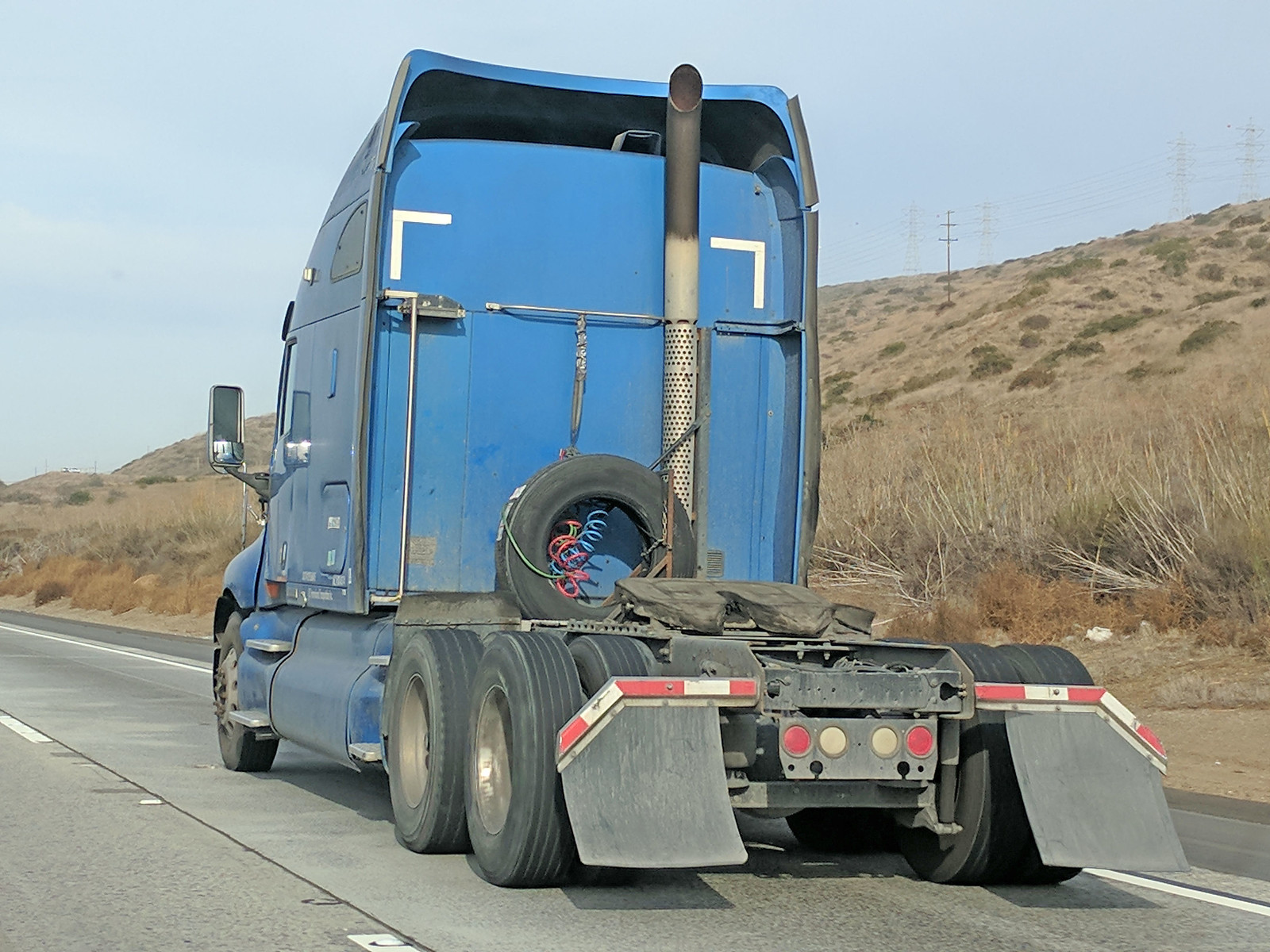This outdoor daytime photograph depicts a three-quarter rear view of a blue semi-truck cab driving along a paved desert highway, likely in the United States. The truck, lacking its trailer, reveals details such as two rear axles, mud flaps with reflectors, and a spare tire secured against the back of the cab. The cab features a prominent air dam, or spoiler, atop and a long exhaust pipe extending upward. The semi-truck is slightly dirty, and there are no identifying logos or text on it. The highway, marked by a broken white line, stretches diagonally from the lower right to the upper left of the image. Surrounding the truck are dry, desert hills with sparse sagebrush and power lines running along the ridges. The sky is a light blue with minimal clouds, contributing to the clear, bright lighting of the photograph.